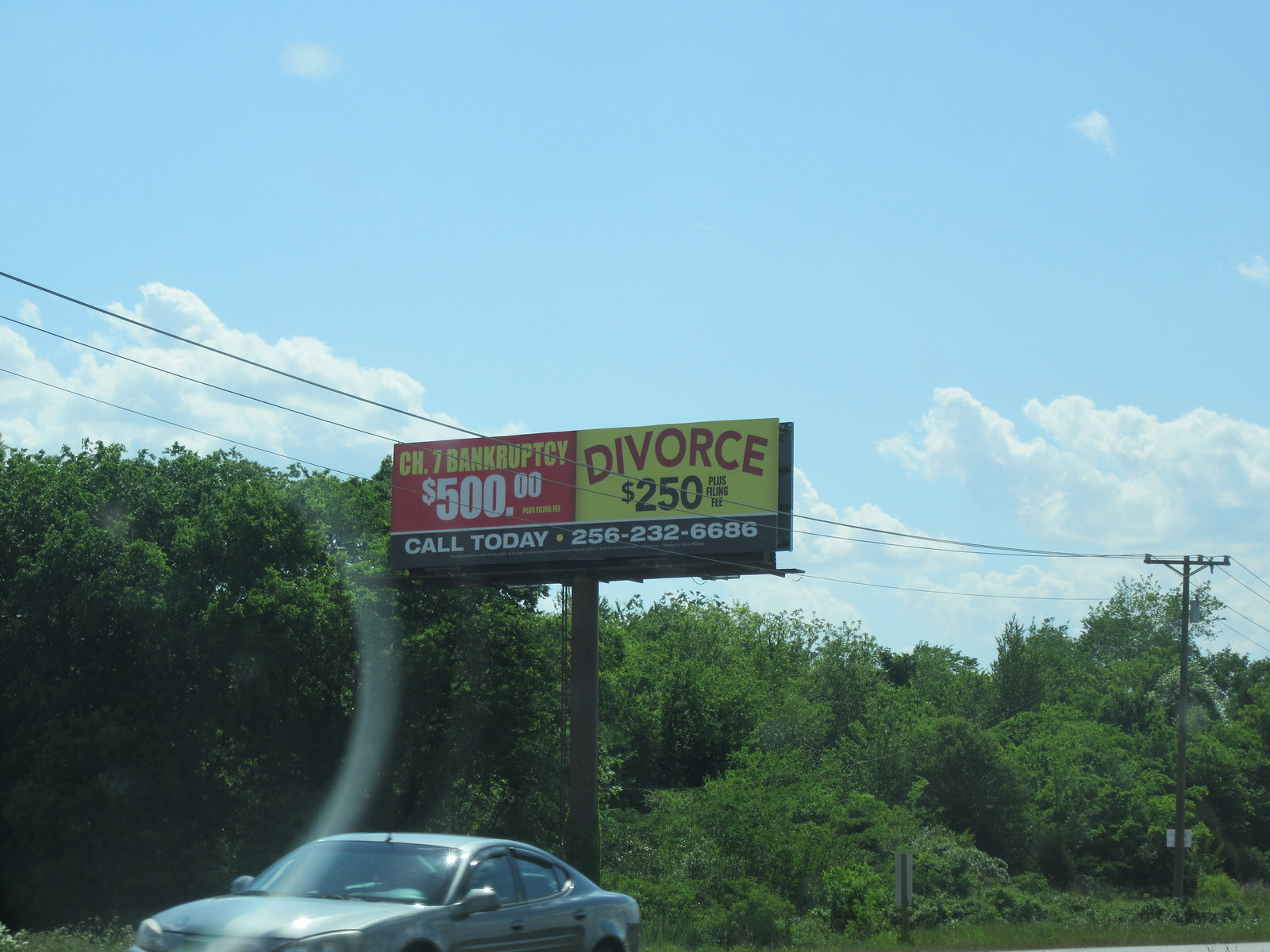In this outdoor nature scene, a photograph captures a roadside billboard towering on a single brown metal pole with a walkway underneath, framed against a vivid blue sky adorned with scattered white clouds. At ground level, a medium-sized silver car drives by on the road, adding a dynamic element to the serene setting. The billboard is divided into two contrasting halves: the left side is red with bold yellow lettering advertising "Chapter 7 Bankruptcy, $500 plus filing fee," while the right side is yellow with red text promoting "Divorce, $250 plus filing fee." At the bottom, a white print urges viewers to "Call Today" followed by the phone number "256-232-6686." A lens flare curls on the left side of the image, enhancing the natural lighting. Behind the billboard, medium-height green trees and lush, tall grass create a verdant backdrop, while power lines run parallel to the road, contributing to the rustic roadside ambiance.